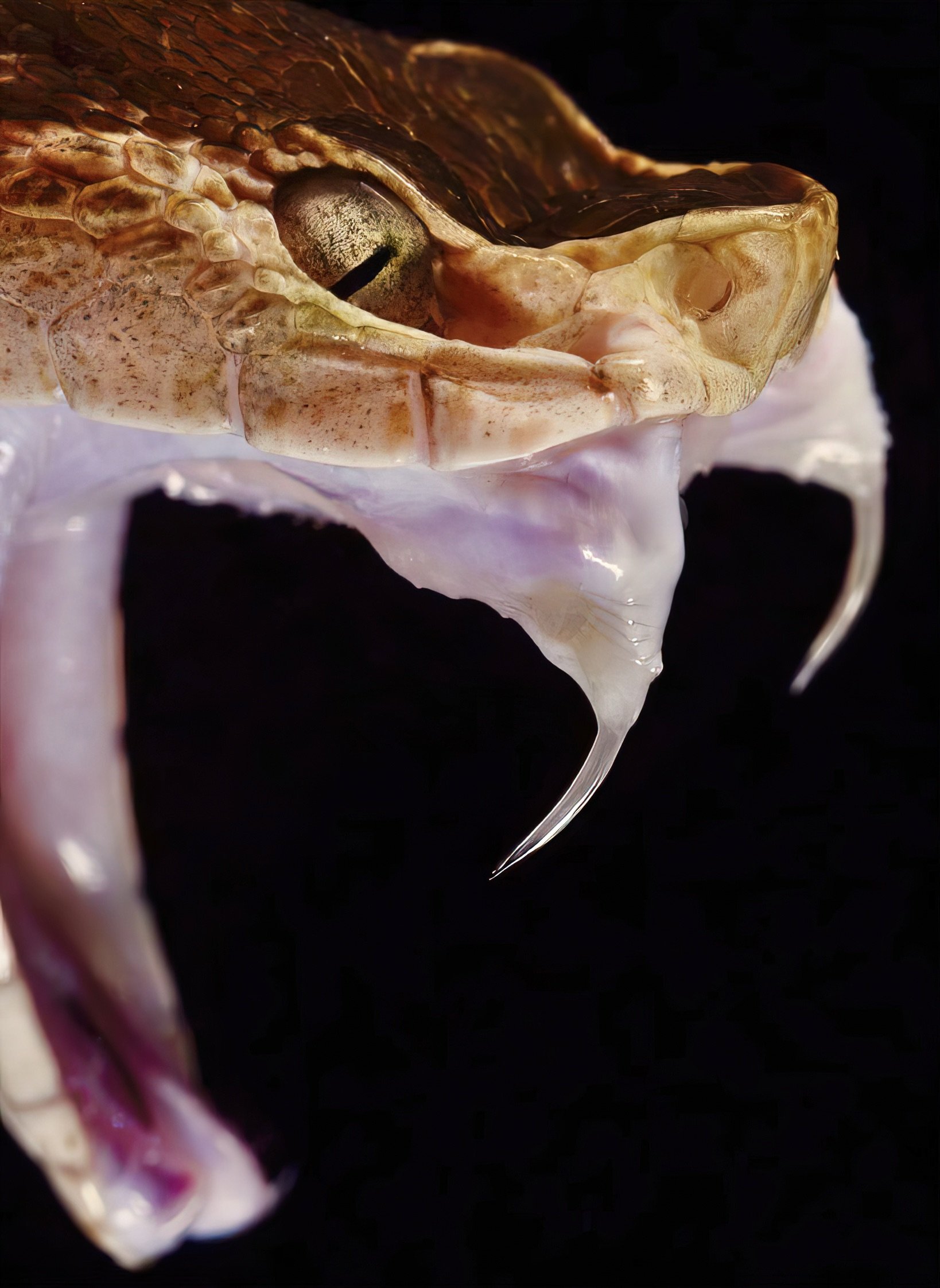This striking close-up photograph captures the fearsome head of a snake, set against a stark black background that accentuates its menacing features. The image focuses on the profile of the snake's head, with its jaw gaping wide to reveal a pale pinkish-purple mouth. At the center of the composition, two prominent, whitish, almost translucent fangs are clearly visible, adding to the sense of danger. The snake's head displays a gradient of brownish-tan hues, with a distinctive darker brown stripe running down the center. One of the snake’s eyes is visible, featuring a vertical, black slit pupil set against a golden iris. This detail, in combination with the pit near its nose, suggests the snake may belong to the Viperidae family, possibly a copperhead, emphasizing its venomous nature.